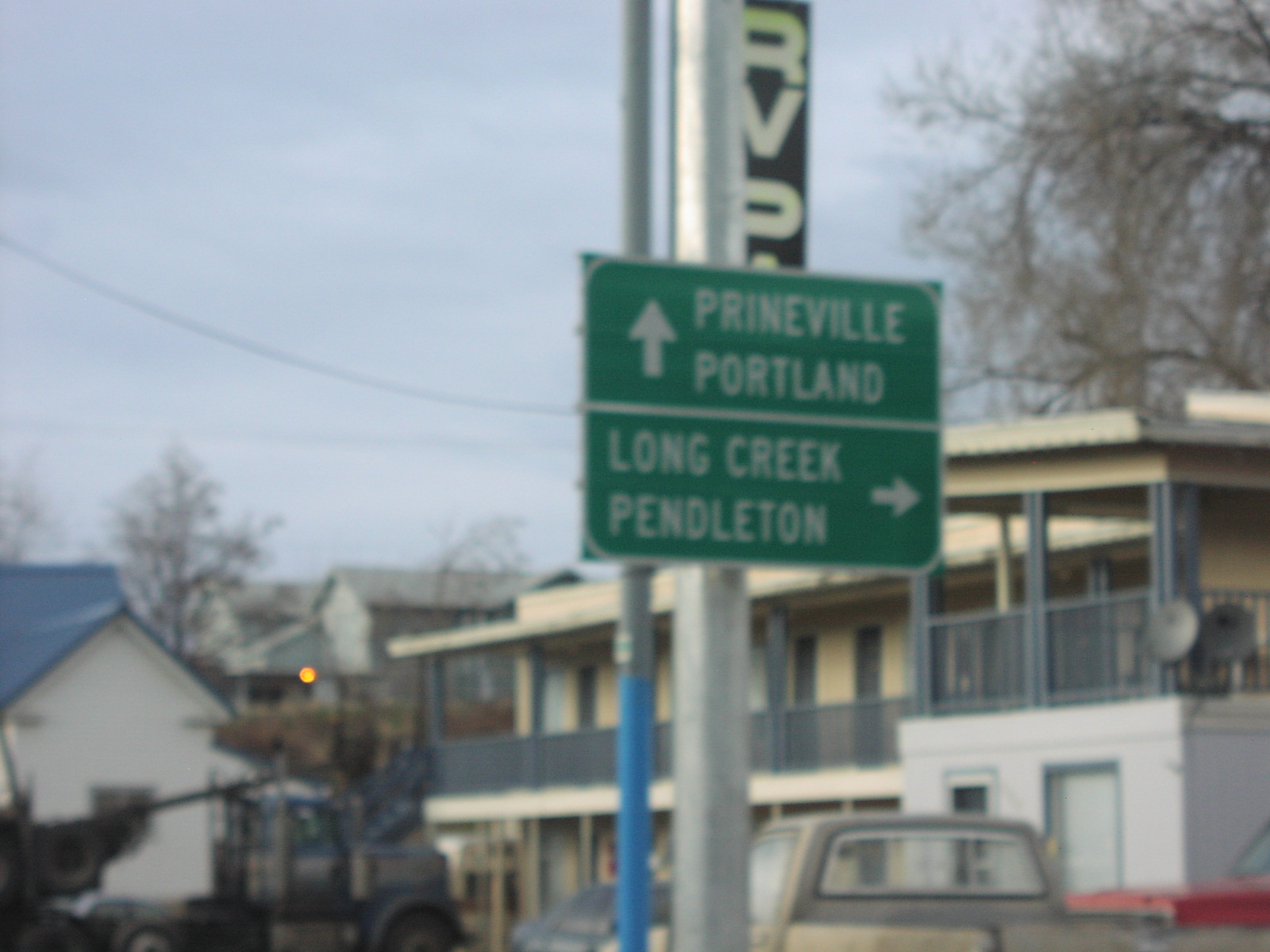The image showcases a concrete structure that could be either a motel or an apartment building. The building features small balconies adjoining each door, lending it a distinctly motel-like appearance. Several satellite dishes are affixed to the exterior, emphasizing its transient or multi-tenant nature. In the foreground, a street sign provides directional information, reading "Straight ahead to Preenville, Portland" and "Long Crete, Pendleton" with an arrow pointing to the right. This reference to Portland suggests that the location might be in Oregon. Adding to the scene's roadside feel are vehicles parked in the lot: a pickup truck and what appears to be the cab of a large truck, supporting the notion that this establishment serves as a convenient rest stop along the highway.